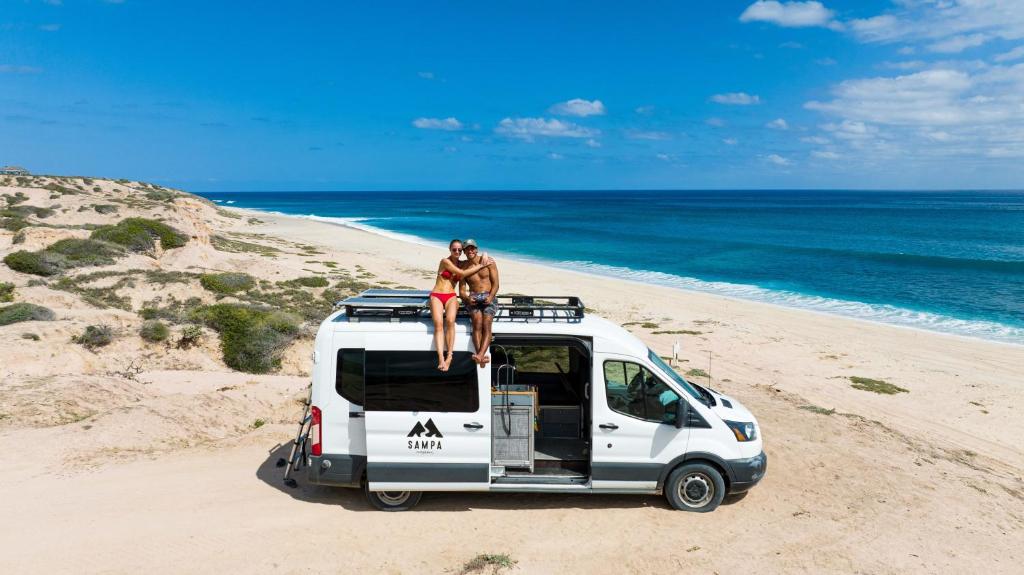The image captures a sunny day at the beach, with a light blue sky accented by a few clouds. The vibrant blue ocean dominates the scene, accompanied by white waves crashing gently on the sandy shore. A white van labeled "Sampa" with a logo of two mountains is parked on the beach with its side door facing the camera open. On top of the van, a man and a woman are sitting on a roof rack, hugging and posing for the picture. Both are in beach attire; the woman is wearing a swimsuit while the man is in swim trunks and a baseball cap, with both sporting sunglasses. To the left of the beach, a hill with sparse grass adds to the natural setting, while the waves on the right side of the image appear calm. The van is oriented towards the right, perfectly framing the idyllic beach scene.